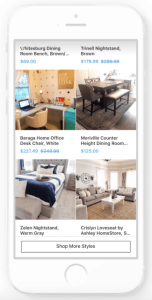This image features a mock-up of an e-commerce furniture website displayed on a white iPhone. The iPhone is an older model, distinguishable by its substantial white plastic borders at the top and bottom, and a central white home button. The phone screen exhibits a drop shadow effect on the side and several buttons on the left.

The display on the iPhone is notably grainy, blurry, and highly compressed, making finer details hard to discern. However, the mock-up showcases multiple interior design shots arranged in a grid format. In the top-left quadrant, there is an image of a desk setup in front of a window, featuring a laptop. Adjacent to this, on the top-right, there's a photograph of a simple dining room set.

The bottom section presents additional furniture: the lower-left quadrant features a bedroom with a bed, while the lower-right quadrant displays a complete living room set. The bottom images are accompanied by a prompt to "shop more styles" but lack visible price tags.

Conversely, the images in the top row include pricing information. The desk set has an original price of $399, which is crossed out and reduced to $2.27 (presumably a placeholder text or formatting error). The specific price for the dining room set remains unreadable.

Above these images, there are further price listings unaccompanied by visuals, suggesting more items available upon scrolling. The mock-up appears to be an early prototype for an app, likely under development.